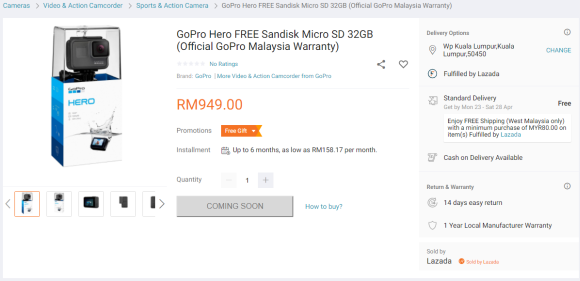Certainly! Here's a more polished and detailed caption:

---

This is a product page on a website for purchasing a GoPro Hero action camera. The top navigation menu includes sections for Cameras, Videos & Action Camcorders, Sports & Action Cameras, and more. The featured product is the GoPro Hero, displayed prominently in its packaging. Surrounding the main image, there are five thumbnails with navigation arrows indicating additional views are available. The box itself is branded with "Hero" and includes an offer for a free 32GB SanDisk microSD card, alongside the assurance of an official GoPro Malaysia warranty.

The listing showcases multiple product details. The price is noted as RM 949, with a promotion offering a free gift. For payment flexibility, installment plans are available for up to six months, starting at RM 158.17 per month. The product is currently unavailable, indicated by a grey "Coming Soon" button. 

Adjacent to the purchasing information, there are delivery options specified for WK Kuala Lumpur, costing RM 54.50, with an option to change the delivery location. This product is fulfilled by Lazada, as stated clearly on the page.

---

This caption provides a comprehensive overview of the web page, enhancing readability and detail.